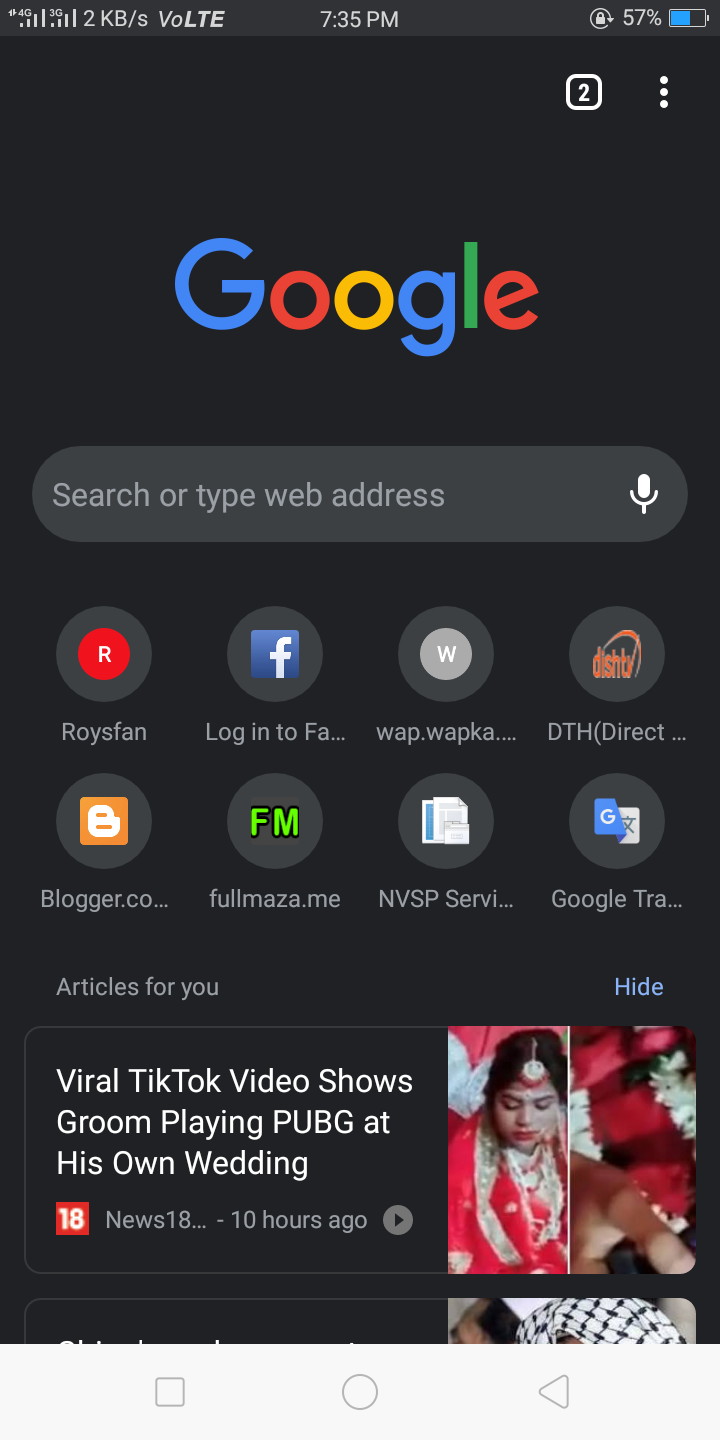**Detailed Caption:**

This image captures a screenshot of the Google search homepage. Prominently centered at the top is the iconic, multi-colored Google logo. Directly beneath the logo lies the familiar grey search bar, inviting users with the text, "Search or type web address." On the right side of this search bar is a small microphone icon, indicating the voice search functionality.

Further down, two rows of circular icons display various bookmarked websites, reflecting the user's frequently visited pages. Each icon is enclosed within a circle. The bookmarks include:

1. "Roy's Fan" – a possible webpage title or username.
2. Facebook login page, denoted as "login to facebook.com."
3. "Wap.wapka" – perhaps a mobile site or service.
4. "BHT" – possibly referring to a specific website or service acronym.
5. "Dish TV" – likely a television service provider's site.
6. "Blogger.co" – a potential blogging platform.
7. "FullNASA.me" – a site possibly related to NASA.
8. "NVSP" – could represent a particular user’s site or service acronym.
9. "Google" – indicative of a direct link to Google services or a related page.
10. "FirstOracleShown" – might be a unique or specific web page title.
11. "Viral TikTok video" – a link presumably leading to a trending TikTok video.

The layout and bookmarks suggest the user's preferences and frequently visited websites, showcasing a blend of personal interests and utility services.